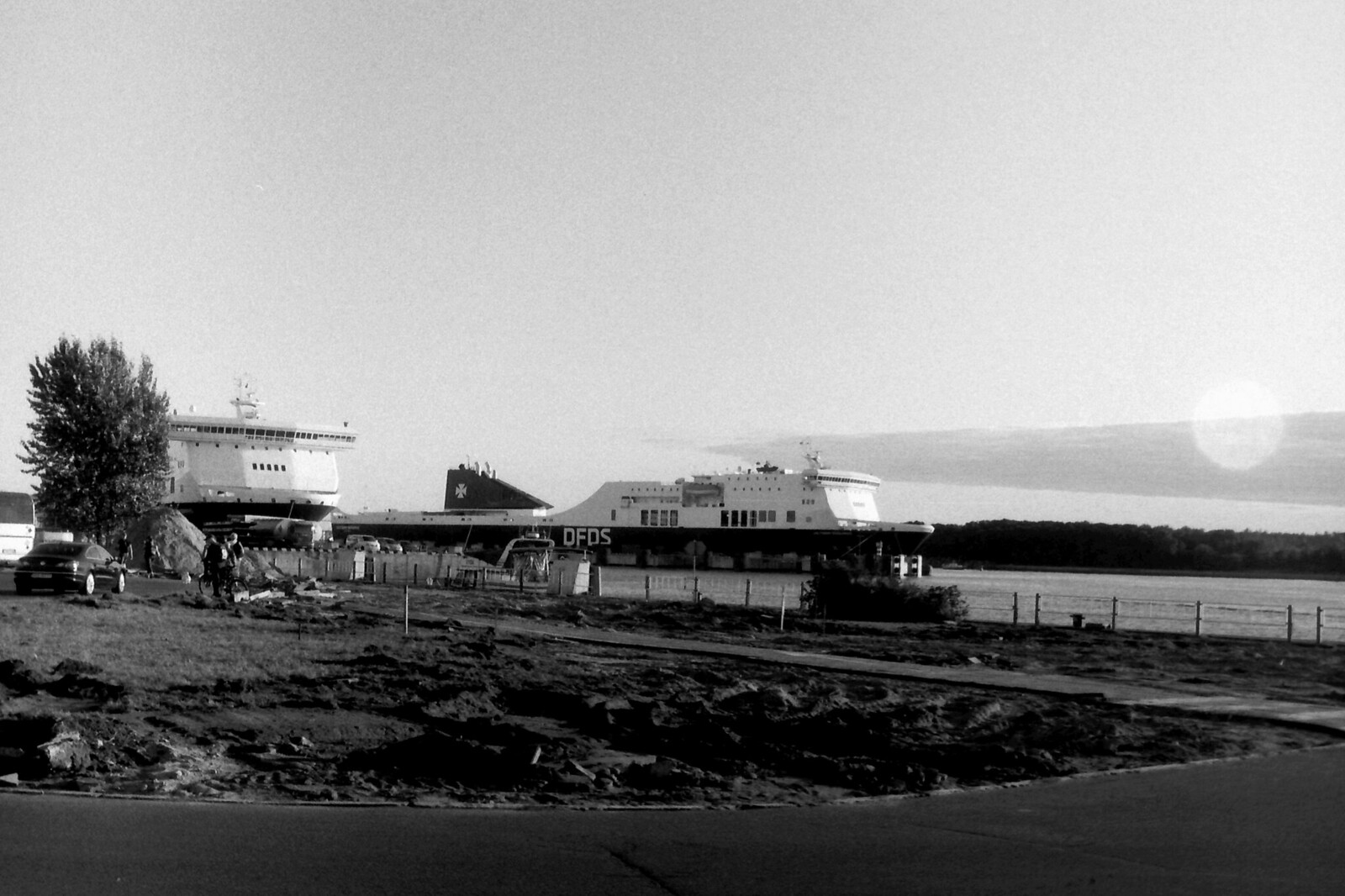The black-and-white vintage photograph captures a detailed outdoor scene dominated by a large ship, presumably a ferry, docked by a body of water, which could be a river or a coastal area. The ship has the letters "BFDS" prominently displayed on its mostly white hull, with some black accents. In the foreground, there is a sidewalk or road that transitions into some unclear terrain, possibly a mix of dirt and mud. To the left side of the image, there is grass, a tree, and a car, as well as a structure that appears to be a building or lookout post. Further back, another sidewalk borders the water, and the setting sun or rising sun casts a low light across the scene, suggesting the time of either sunrise or sunset. Beyond the ship and water, there's a line of trees against a plain sky, contributing to the serene atmosphere of this timeless capture.